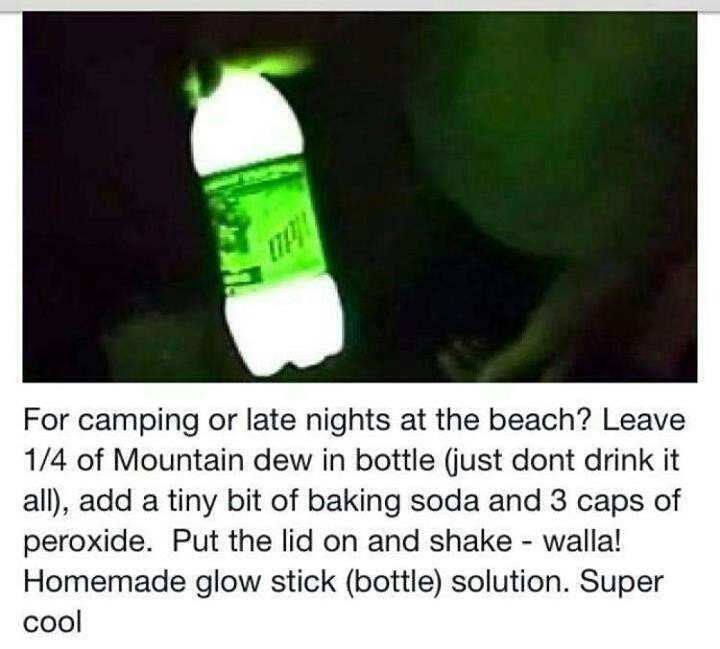The image depicts a glowing Mountain Dew bottle held by a hand, set against a very dark and blurred background. The bottle emits a bright light, illuminating its green label, though the text on the label is unreadable due to the image quality. The hand, partially visible, grips the bottle from the top, while the surrounding darkness suggests a night scene, possibly indoors. Above the image, a thin gray border spans horizontally. Below the image, text explains that this is a DIY glow stick bottle for camping or late nights at the beach. The instructions detail: leave a quarter of Mountain Dew in the bottle (not to drink it all is emphasized), add a tiny bit of baking soda, three caps of peroxide, then put the lid on and shake to create this glowing effect. The text is arranged in five lines and describes the concoction as a 'super cool' homemade solution.